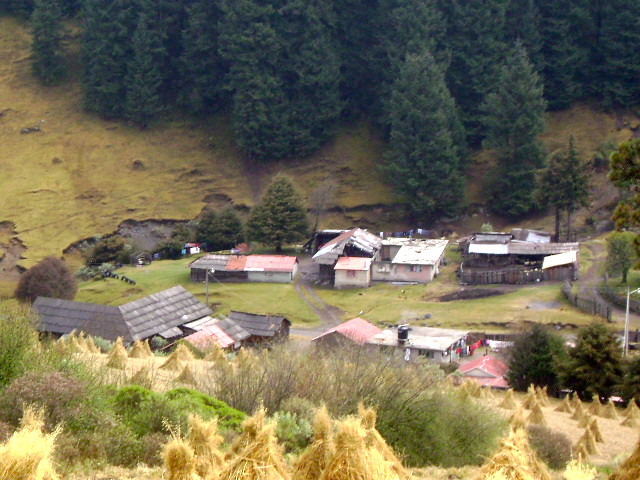This photo captures a picturesque small village nestled in a verdant valley, surrounded by rolling hills and dense, dark green evergreen trees. The image, taken from a hillside vantage point, reveals six or seven houses flanking a central dirt road that meanders through the village. Unique fences and shrubbery accentuate the homes, which feature a mix of red roofs and white or gray exteriors. In the front yards and behind some homes, clotheslines with hanging laundry hint at daily life. Below a steep, forested hillside, the scene is dotted with patches of yellowing trees and pyramids of hay, indicative of farmland. The natural setting — abundant with pine or fir trees, tan and green shrubs, and grassy fields — suggests a serene, rural environment captured vividly under daylight conditions.